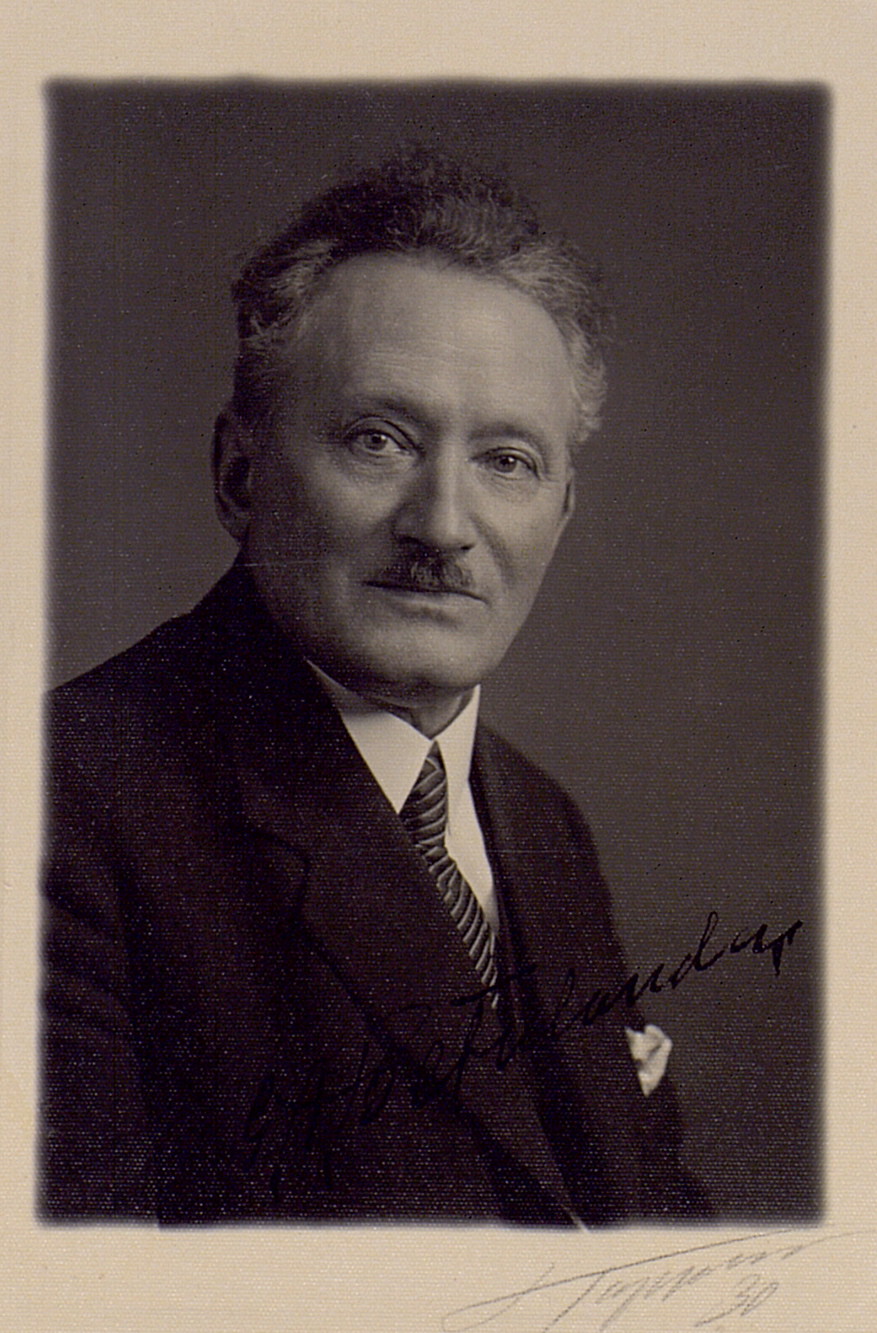The photo is a black-and-white, possibly sepia-toned portrait of an older gentleman, likely in his 60s, with graying hair styled upwards. He wears a dark suit paired with a white collared shirt and a striped tie. A neatly folded handkerchief peeks from his breast pocket. The man, who appears to be sitting and looking slightly over his shoulder towards the camera, sports a small mustache that extends from the center of his nose to just short of the corners of his mouth, maintaining a neutral, straight-lipped expression. The background of the photo is dark gray, and the image is affixed to a lighter gray or white canvas-like backing, suggesting the photo might have been airbrushed or copied. There are two signatures: one located near the handkerchief pocket and another, written in pencil, at the bottom on the canvas, both featuring the number "30," suggesting the photo might date back to the 1930s or 1940s. The subject's eyes seem to be brown, although it's challenging to discern precisely. The overall aesthetic of the portrait gives it a vintage, well-preserved quality.